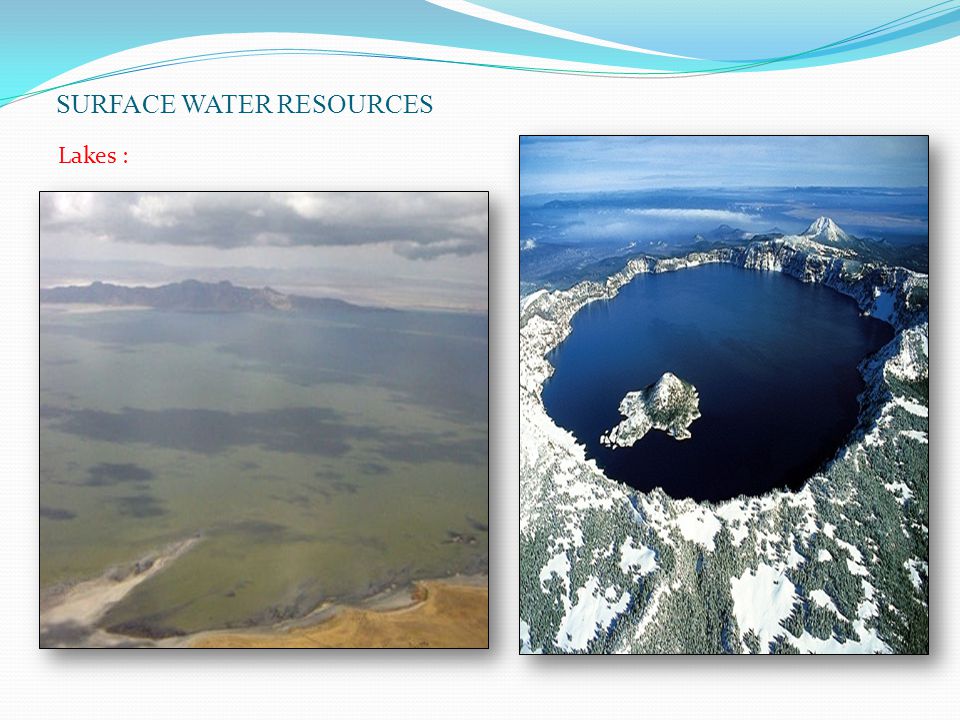The image features an infographic titled "Surface Water Resources" with two color photographs under a decorative blue computer graphic at the top. It showcases aerial views of high-altitude lakes and is formatted against a clean, white background with a light blue ornamental design across the top.

The first photograph on the left, slightly smaller and square-shaped, captures an aerial view of a valley with a mountain range and a large body of greenish-blue water reflecting the clouds above. The shore of this lake is sandy and golden-colored, with green grass valleys and a mountain range in the distance under a sky dotted with clouds.

The second photograph on the right, taller and in portrait orientation, depicts an alpine lake bordered by snow patches, situated above the cloud line with a clear blue sky and distant landscape visible. Both images are bordered by thin black lines and clearly spaced side-by-side, suggesting a presentation-style layout that might have been designed using PowerPoint. The headings "Surface Water Resources" and "Lakes" are prominently displayed in dark blue and red typography respectively, enhancing the informative and visual appeal of the infographic.